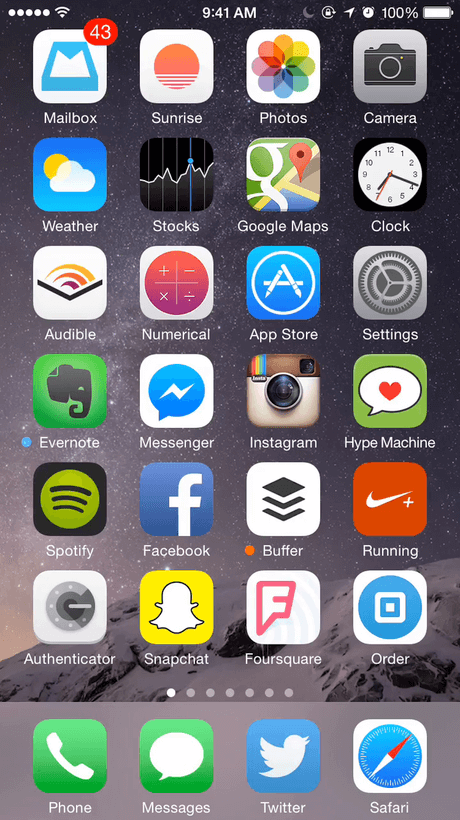This is a detailed screenshot of an iPhone home screen, showcasing various elements and icons. At the very top, there are five white dots indicating full signal strength, followed by a full Wi-Fi symbol. In the center, the time 9:41 AM is displayed in bold. Surrounding the time are several icons: a quarter moon symbol indicating "Do Not Disturb" mode, a lock symbol, an arrow symbol showing location services are active, an alarm clock symbol, and a fully charged battery icon.

The home screen itself consists of six rows of application icons, with four icons in each row:

1. **First Row**: Mailbox, Sunrise, Photos, Camera
2. **Second Row**: Weather, Stocks, Google Maps, Clock
3. **Third Row**: Audible, Numerical, App Store, Settings
4. **Fourth Row**: Evernote (with a blue dot next to it), Messenger, Instagram, Hype Machine
5. **Fifth Row**: Spotify, Facebook, Buffer (with an orange dot next to it), Nike+ Run Club
6. **Sixth Row**: Authenticator, Snapchat, Foursquare, Order

Below these rows, seven dots indicate multiple screens available for swiping. At the bottom is a gray dock containing four essential apps: Phone, Messages, Twitter, and Safari.

The background of the home screen is an awe-inspiring image of a starry night over a snowy mountain peak, with dark gray and black rocks emerging through the snow, adding to the serene ambiance.